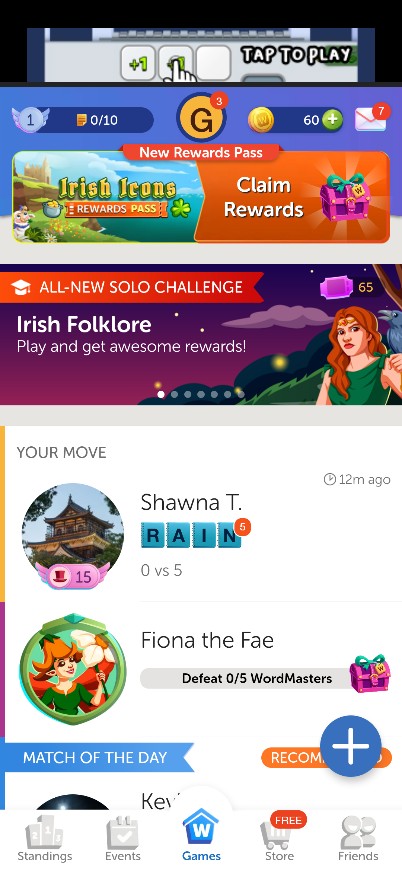**Descriptive Caption:**

This is a detailed screenshot taken from a smartphone, showcasing a menu from a mobile game. The image is portrait-oriented, comprising several distinct sections stacked vertically.

At the very top, there is a thin black bar occupying approximately 10% of the screen. This bar features a small advertisement with partially visible text saying "Tap to Play" and a small cursor pressing buttons. 

Below this, a section that takes up about a quarter of the screen displays a dark blue to purple gradient background, serving as an advert for "Irish Icons." Within this section, there is an orange highlighted box with white text saying "Claim Rewards" and a purple treasure chest illustration to its right. Next to it, in yellow, the text reads "Irish Icons," with "Rewards Pass" in white text on an orange rectangular background underneath it. The background of this section also includes a cartoon drawing of a church on a cliffside overlooking the ocean. Above these elements, a silver circular box indicates the user has 0 out of 10 rewards and is at level 1. In the middle, a yellow circle with a black arrow features a notification marked by a smaller orange circle with the number 3. To the right, a small dark blue pill box contains the number 60 in white text, next to a green circle with a white plus symbol. Additionally, there is a mail icon with the number 7 in an orange circle in the corner.

The next section, occupying roughly a third of the screen, contains another advertisement. This section includes a light to dark orange banner stating "All New Solo Challenge" in white text. Below this, the main body of the advert, in white text, reads "Irish Folklore, play and get some awesome rewards." The background features a cartoon drawing of a woman with a crow on her shoulder, standing on a hillside and frowning into the camera. An indicator above her shows the number 65 next to a pink ticket illustration. The sky behind her transitions from dark purple to light purple, suggesting dusk.

The final section reveals part of the actual game menu on a white background. In the top left corner, it says "Your Move" in black text. Along the left border, a yellow line transitions into equal portions of purple and blue. Below "Your Move," a circle shows a cartoon Asian-styled house. Adjacent to this, a small pill-shaped box containing the number 15 and a hat symbol belongs to "Shauna T," whose name appears in black letters. In blue squares below this, the word "Rain" is spelled out, featuring the number 5 in an orange circle next to the letter "N." Above this box, it states "12M ago" along with a clock symbol in black text.

Further down, it reads "Fiona the Fae," with a grey pill-box stating, "Defeat 0 out of 5 wordmasters" in black text, ending with a dark purple treasure chest adorned with a green bow. "Fiona the Fae" also has a profile circle with a light green border depicting a cartoon woman wearing a dark green dress and a large flower hat. She holds a daisy, partially obscured by the border.

Halfway down this section, a blue banner says "Match of the Day" in white text. To its right, a blue circle with a white plus sign appears alongside a partially visible, orange-bordered "Recommended" banner in white text. 

At the very bottom of the image, a white menu bar with grey symbols is shown, listing "Buildings," "Events," "Games," "Store," and "Friends" from left to right. The "Games" icon is highlighted in blue, featuring a house with a "W" above it.